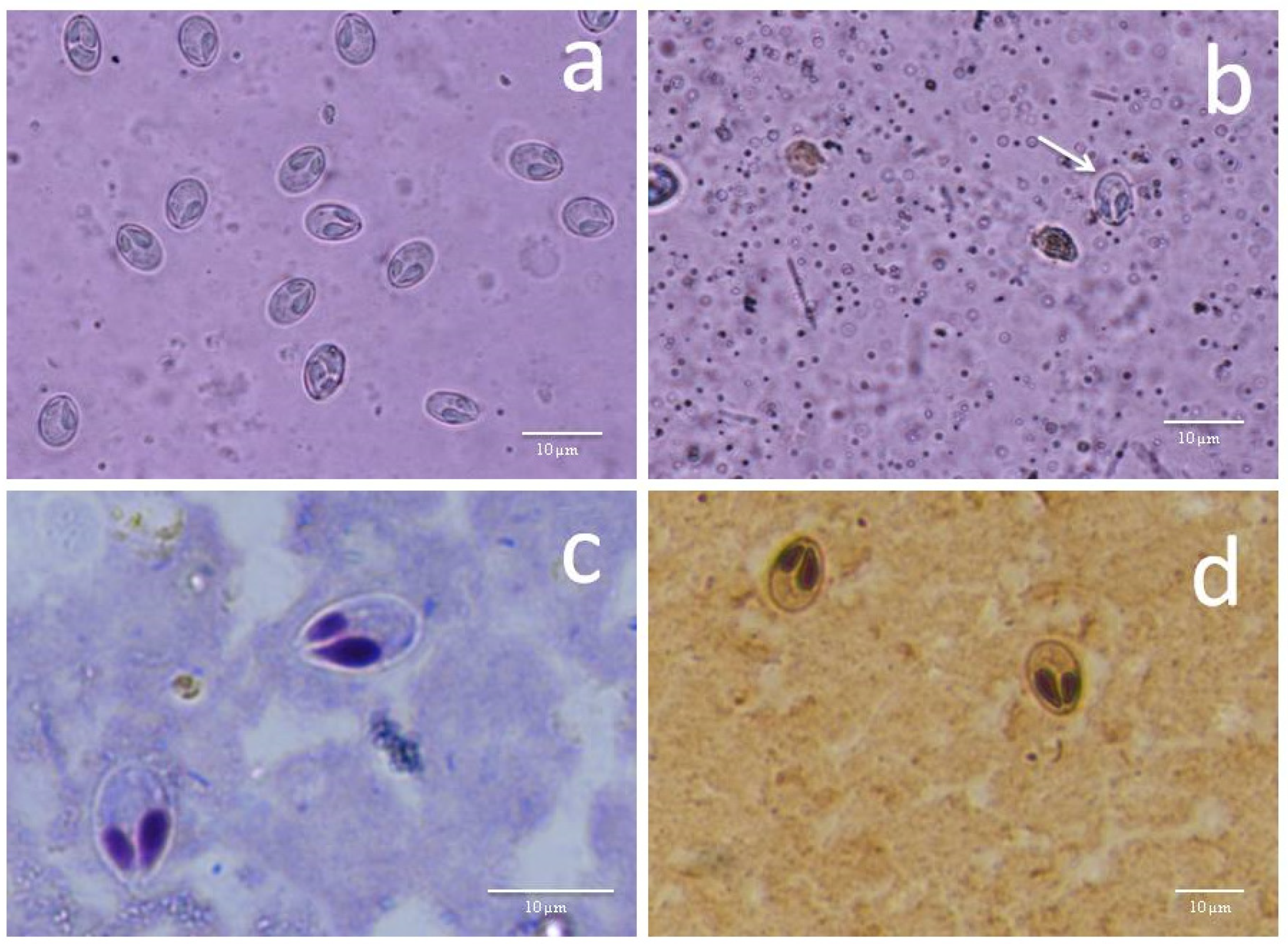The image is a horizontally aligned rectangle that is divided into four sections, each separated by a white border in the form of a cross. These sections are labeled A, B, C, and D in the upper right corner of each sub-image. In the lower right section of each image, there's a horizontal white line indicating a scale of 10 micrometers. 

In section A, located in the upper left quadrant, the background is purple and populated with numerous black oval shapes containing intricate designs inside, resembling cells. Section B, in the upper right quadrant, also has a purple background and features many tiny dark dots, with a white arrow pointing towards a single oval shape similar to those in section A, highlighting it for closer inspection.

Section C, in the lower left quadrant, displays a bluish-gray background and contains two large ovals with smaller, purple-teardrop-shaped inclusions inside, presenting a close-up view of the structures seen in A and B. Finally, section D, in the lower right quadrant, features a light brown background with two brown oval shapes housing black teardrop-shaped inclusions, providing yet another variation of the cellular structures.